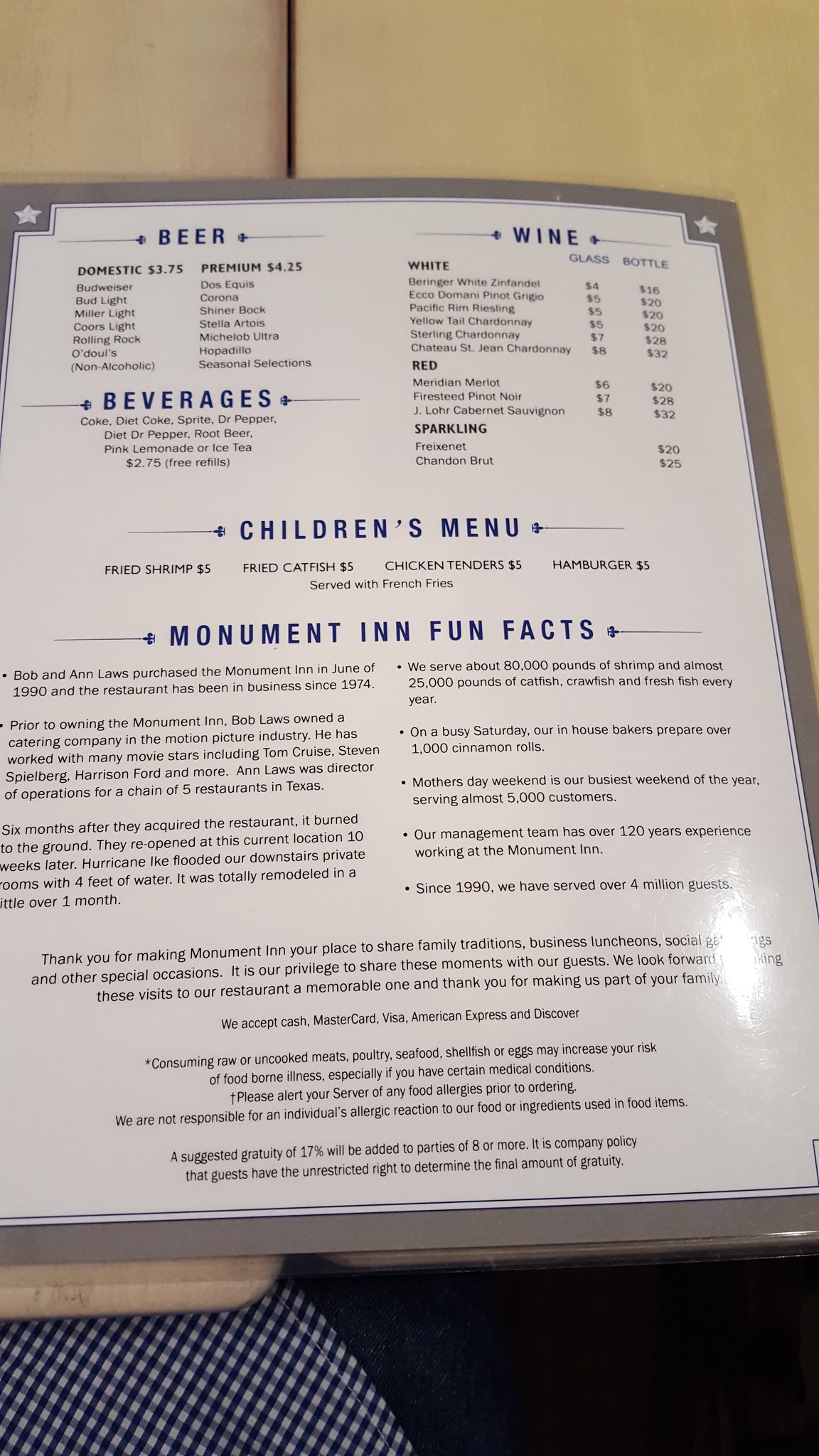The image depicts a close-up of a tabletop with a laminated white menu that has a grey border adorned with white stars at each corner. The menu, illuminated by overhead light, is shiny with significant glare that makes the text mostly illegible. Only the sections labeled "Beer," "Wine," "Beverages," and "Children's Menu," written in blue, along with a bottom section titled "Monument Fun Facts," are discernible, although specific details remain unreadable. The tabletop appears to be formed by two tables pushed together, evidenced by a visible seam between them. At the bottom of the frame, a fragment of a person's attire—a blue and white checkered shirt above blue jeans—is visible, indicating they are seated at the table, engrossed in the menu.